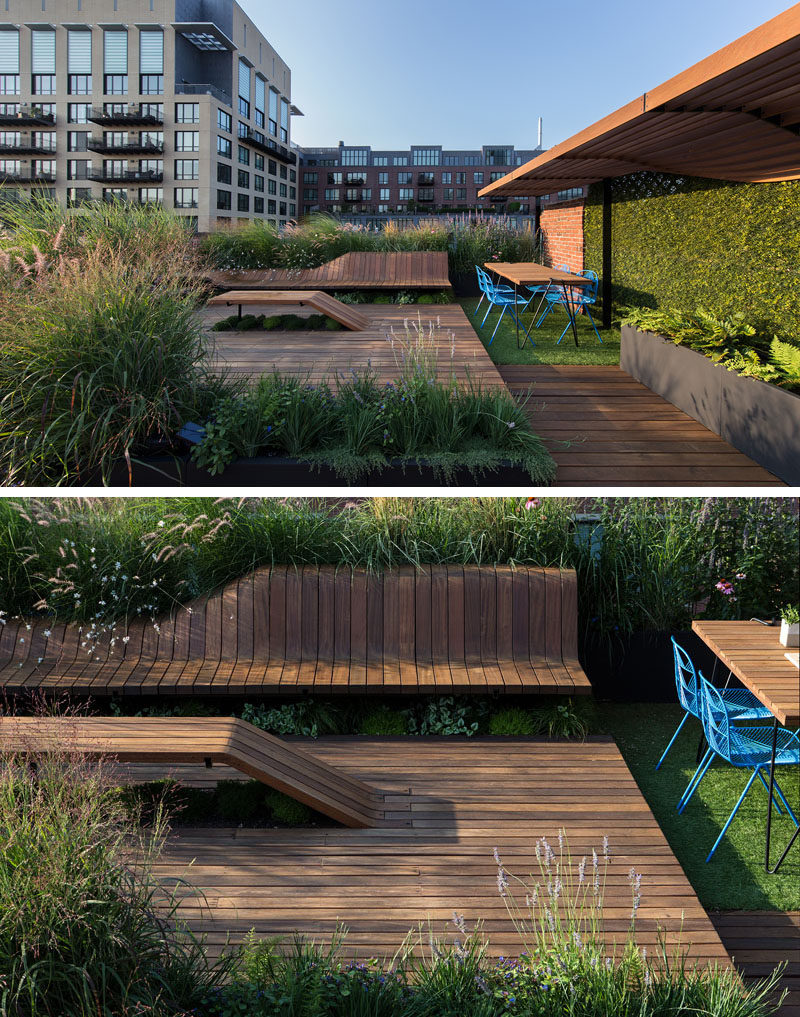The image is a collage of two vertically stacked rectangular photographs depicting an elegant rooftop outdoor space. The top image features a multi-storied grey building, likely an apartment complex or factory, serving as the backdrop. In the forefront, there's an outdoor setting adorned with a variety of garden furniture, including a long brown wooden bench, a dining table with blue chairs, and an assortment of wooden structures. The area is paved with dark brown wooden floors, showcasing their natural texture. To the right, there is a covered section with a red roof, and beyond it, a green wall lush with plants and ferns. 

The setting is surrounded by an abundance of greenery, including bushes, hedges, and specific plants like lavender, creating a verdant and inviting atmosphere. The bottom image is a close-up of this same rooftop space, highlighting the wooden deck and garden furniture in more detail. Here, the details like the blue chairs around the dining table, a patch of grass behind the bench, and the various plants are more prominent, providing a clearer view of the texture and arrangement in this tranquil urban oasis.